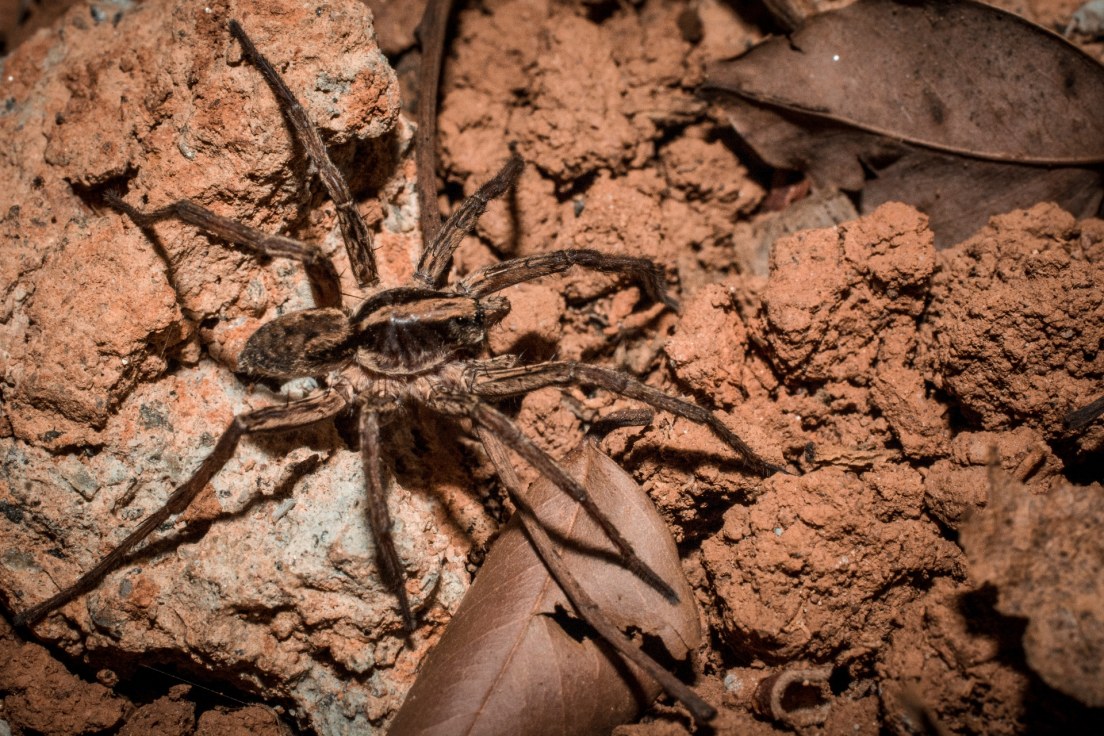The photograph is a detailed macro shot taken outdoors, capturing a large, brown, and very hairy spider with black markings. The spider's body features a distinct light brown stripe down the center and darker black smudges on the sides, with a small brown patterned abdomen. It is seen crawling across a terrain that's a mix of brown, dusty rocks, and grayish rocks resembling dried mud. The environment also includes dead, brown leaves—one prominently underneath and to the lower right of the spider, and another in the top right corner of the image. The entire color scheme of the photograph is dominated by shades of brown and gray, emphasizing the earthy, natural setting. The spider's eight legs are widely spread as it navigates the rugged, leafy terrain.